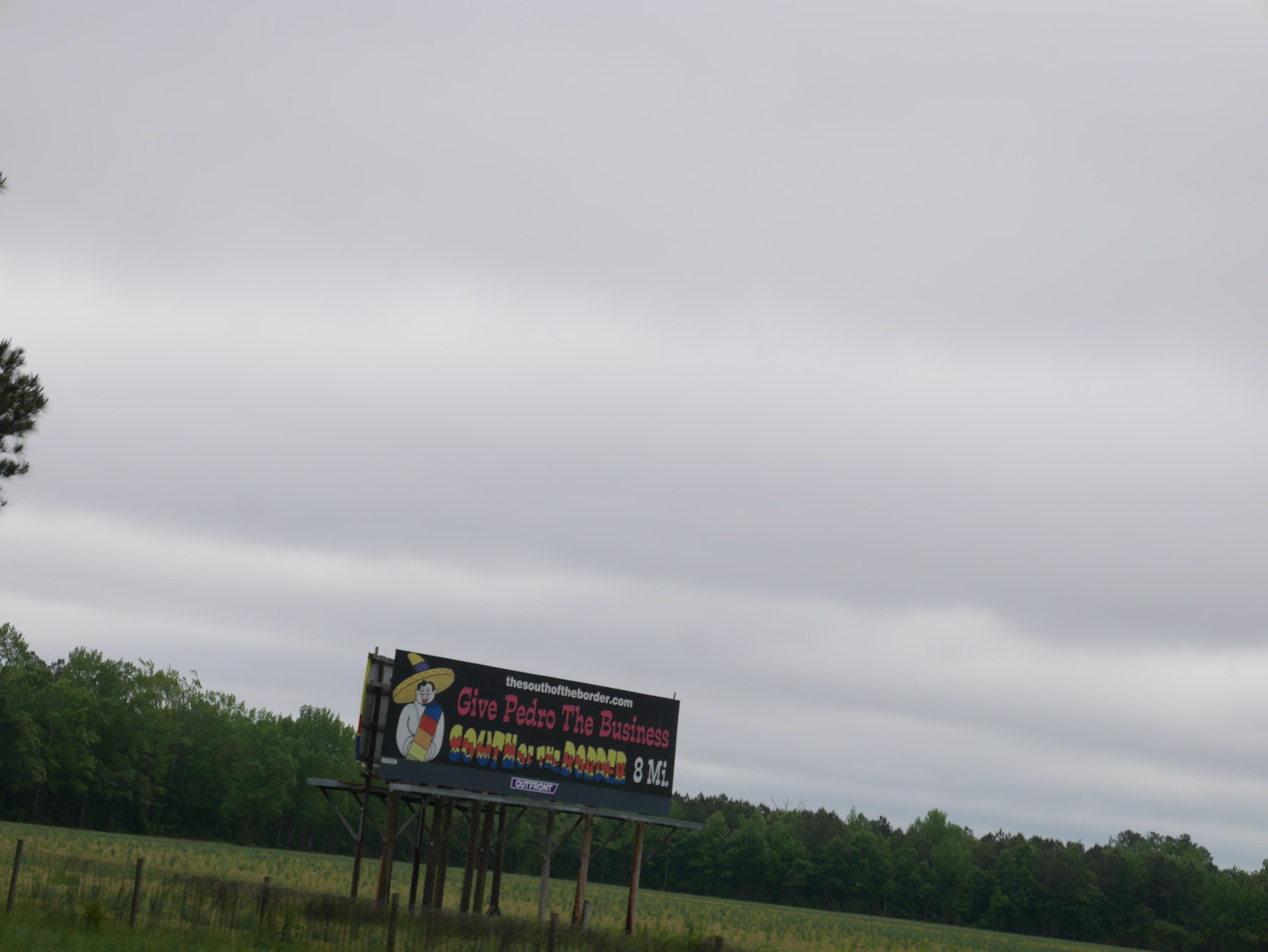This color photograph showcases a predominantly grey sky, occupying about 80% of the frame. The distant horizon is slightly slanted, suggesting the camera was tilted approximately 45 degrees to the right during capture. In the background, a hedgerow of trees lines the horizon, with the edge of a larger tree visible on the extreme left. Below this tree, patches of green grass are evident.

To the left of the center, a platform supported by numerous thin legs stands prominent. The platform features a rectangular sign with a black background. The sign's left side displays a cartoon figure wearing what appears to be a wide-brimmed hat, possibly a sombrero. The character has a white head and body and is adorned with a multi-colored scarf in blue, red, and yellow hues. Pink text, difficult to decipher, is positioned next to the figure, accompanied by thinner white text above it which is also hard to read. Additionally, multi-colored text matching the scarf's colors is present below, with some white text on the right side. At the bottom middle of the sign, there is tiny white writing that appears to be part of the sign's display or branding.